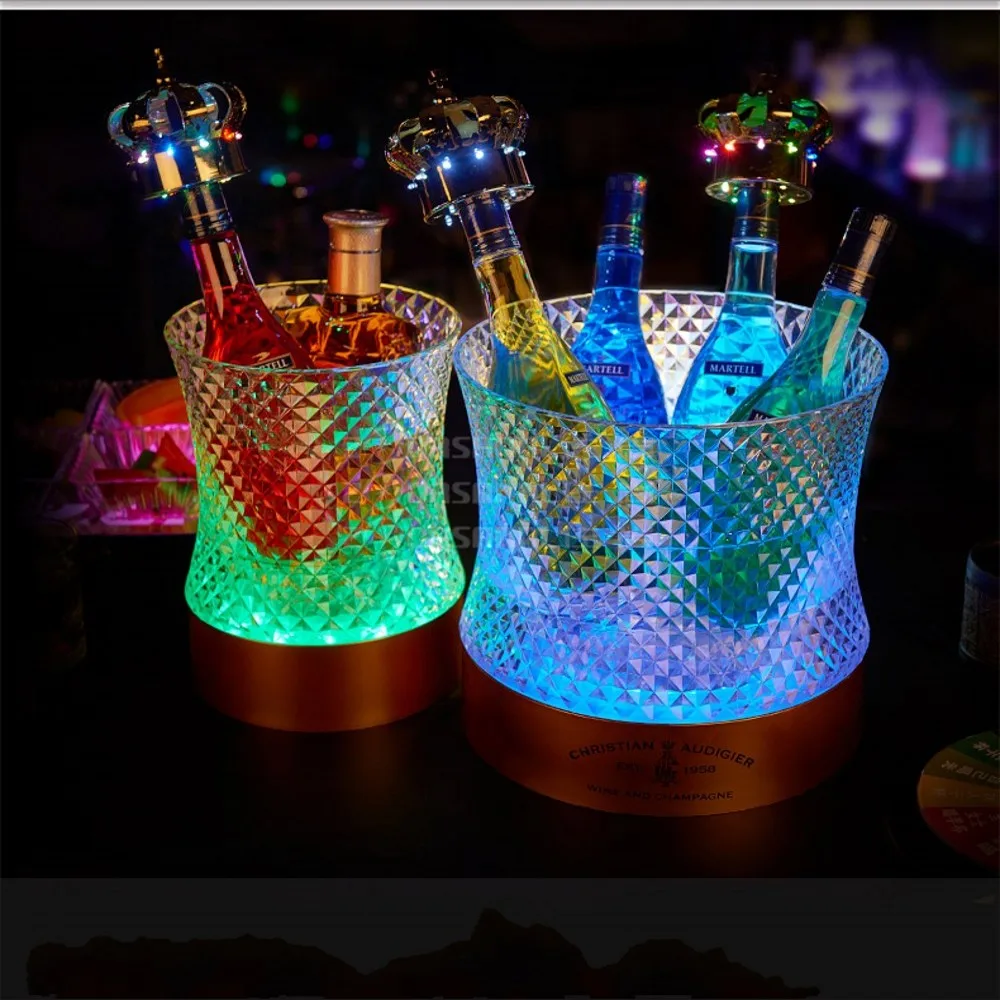The image captures a glamorous scene inside a dimly-lit dance club. The focal point is an elegant bottle service setup featuring an assortment of illuminated designer alcohol bottles, primarily from Martel, positioned in opulent see-through crystal containers. These containers resemble either wine buckets or ice buckets, each adorned with brass bases that bear the inscription "Christian Audigier, 1959, champagne." The bottles inside the containers come in a variety of colors, including brown, yellow, blue, blue-green, and green. Each bottle is topped with ornate stoppers that resemble crowns embellished with lights and jewels, contributing to a neon, glow-in-the-dark atmosphere. The scene behind these opulent containers is dark, enhancing the vivid blue, yellow, red, and orange hues that the bottles emit, making the setup look incredibly fancy and luxurious. Additionally, a spinning wheel, reminiscent of a game of chance with different prizes, is placed next to this elegant display, adding an element of intrigue and entertainment to the sophisticated setting.